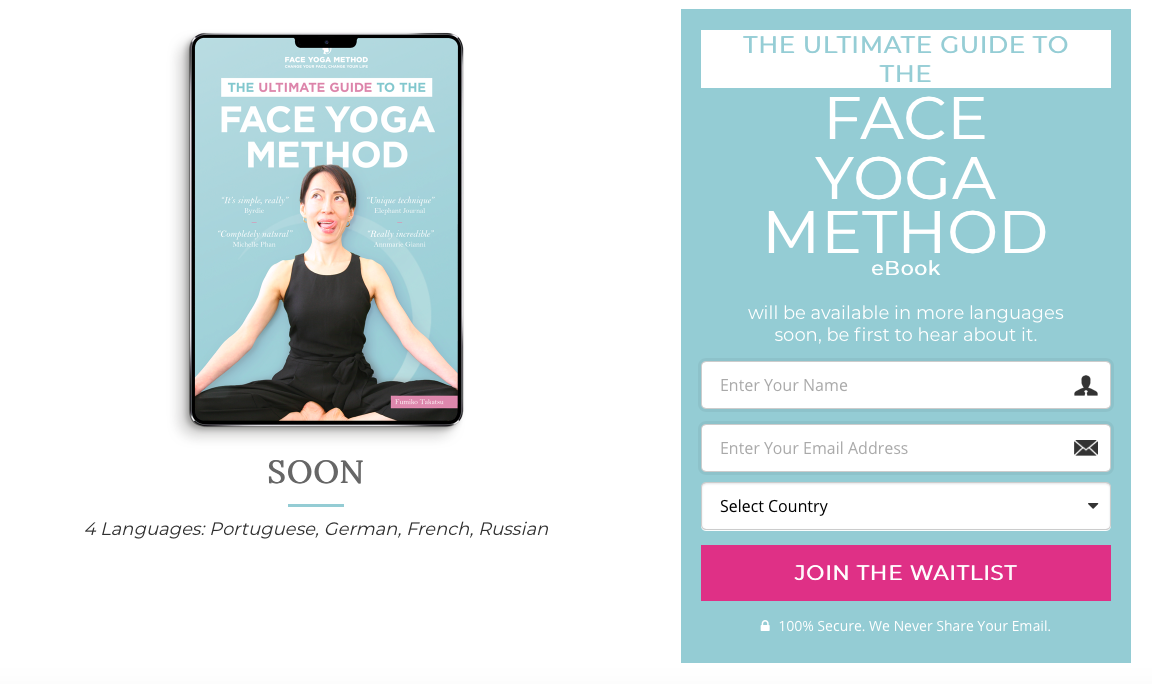The image is a detailed advertisement for a yoga service specializing in face yoga. It features two main sections side by side. 

On the left, there is a photograph of a tablet, likely an iPad, displaying a full-screen image of a woman practicing face yoga. The woman, dressed in black leggings and a black tank top, is seated in a traditional Indian pose. She is performing an exaggerated facial exercise—looking up to her right while extending her tongue to the left as high as possible. Above the image, the text reads, "The Ultimate Guide to the Face Yoga Method."

On the right side of the advertisement, a vibrant sign-up section invites potential customers to join the waitlist for the guide. The headline "Soon in 4 Languages" is displayed in black text, albeit with a typographical error in the word "Portuguese," alongside the names of the languages - German, French, and Russian. 

Below this headline, a light blue section provides spaces for users to enter their details, including their name, email address, and country. A pink button labeled "Join the Waitlist" completes the sign-up form, encouraging immediate action from interested users.

The overall design of the advertisement aligns with modern aesthetic principles, combining relevant imagery with a clear call-to-action to attract and engage potential customers.